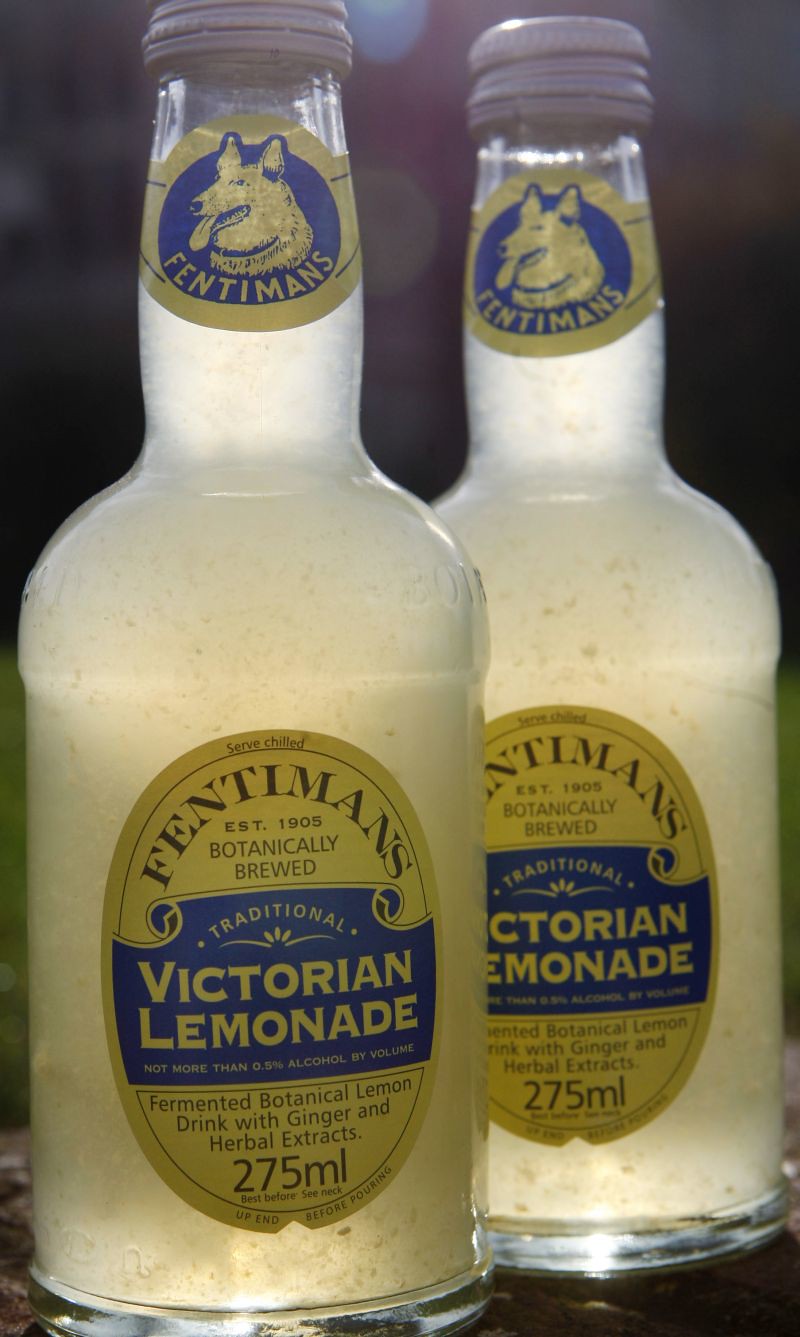The image is a close-up photograph of two glass bottles containing a whitish-yellow liquid with some floating bits inside. Both bottles have twist caps and feature detailed labeling. Around the neck of each bottle, there is a gold label displaying a blue circle with a gold wolf emblem and the text "Fentimans" in gold font beneath it. On the body of each bottle, there is a large oval sticker. This sticker includes various details, such as "Fentimans" at the top, followed by a blue box that reads "Traditional Victorian Lemonade." Additional text on the label mentions "Botanically Brewed," "No more than 0.5% alcoholic volume," and "Fermented Botanical Lemon Drink with Ginger and Herbal Extracts." The bottom of the label indicates the volume as "275 milliliters" and provides instructions like "Serve chilled," "Best before: see neck," and "Up end before pouring." The text on the oval label is primarily in a greenish color, set against a blue background and placed on a black background in the photograph.